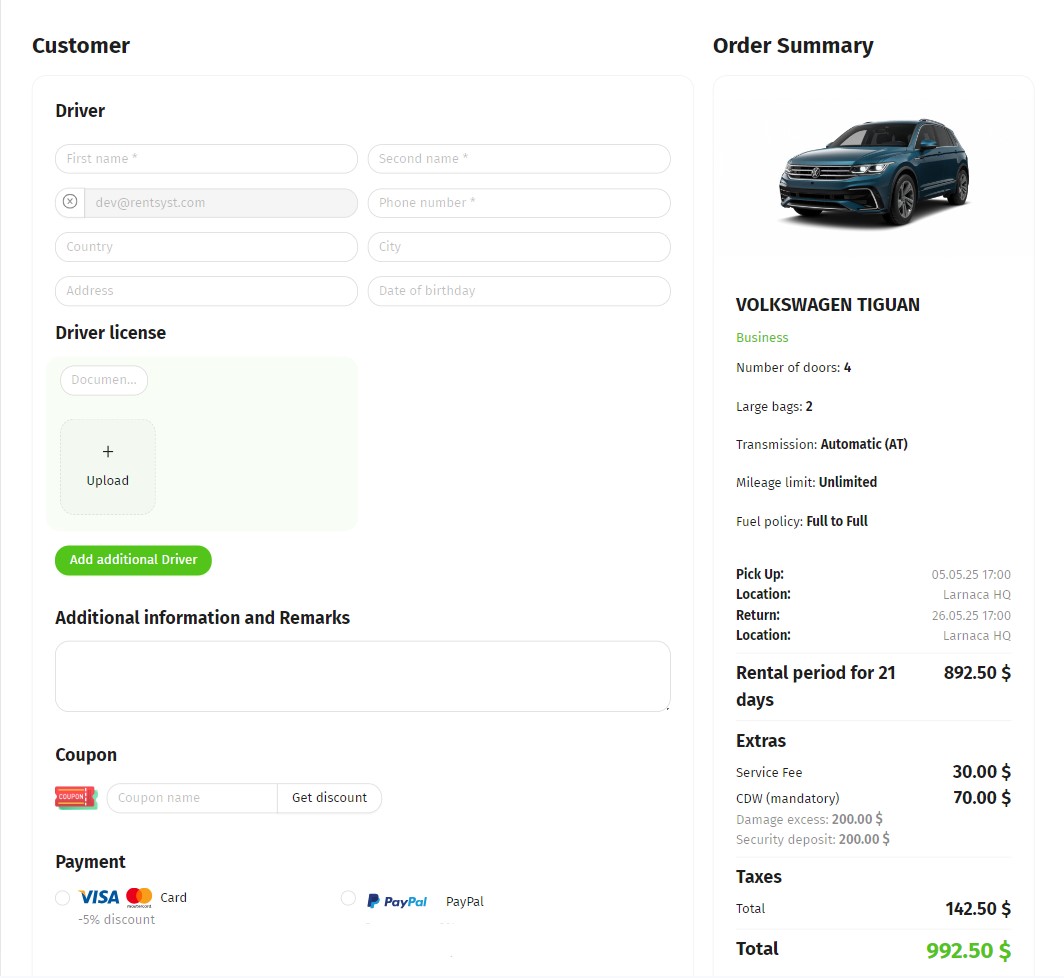Screenshot of a rental car booking page for a Volkswagen Tiguan on a car rental site. The vehicle is categorized under 'Business' class and features four doors and large airbags. The cost breakdown includes a base total of $892.50, with additional extras amounting to $30 and $70, and a service fee of $142.50, bringing the complete total to $992.50. The order summary is displayed on the right side, with a heading in black. The payment fields are currently blank. On the left side, there's a section for driver information, which is also blank, labeled 'Customer.' A green button labeled 'Add Additional Driver' is present, indicating the option to include another driver.